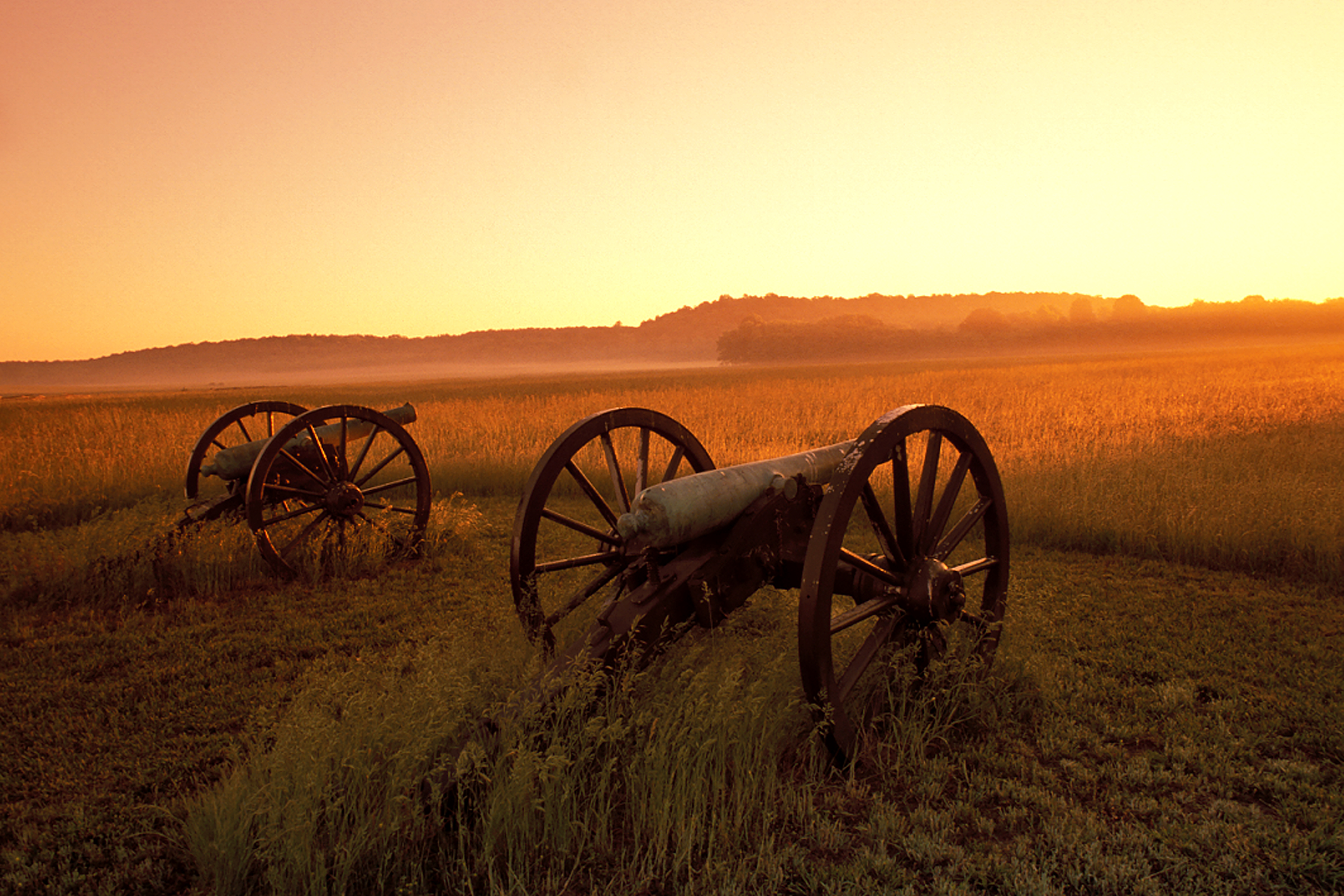In this outdoor photograph, there are two old Civil War-era cannons situated prominently in the middle of a level, grassy field. Each cannon features two large, brown, wooden wagon wheels, with the gray cannon barrel centered between them. The cannons are aligned side-by-side and both are aimed toward the top right corner of the image. The field in which they stand is a mix of tall, green and brown grasses that give the setting a somewhat rugged appearance. In the background, you can see more tall grasses illuminated by the setting sun, which casts a golden hue over the distant landscape, including a range of indistinct trees or possibly low hills. The sky exhibits a gradient of colors from a bright, light orange on the right side, where the sun is setting, to a reddish tone on the upper left side, adding a warm glow to the entire scene.